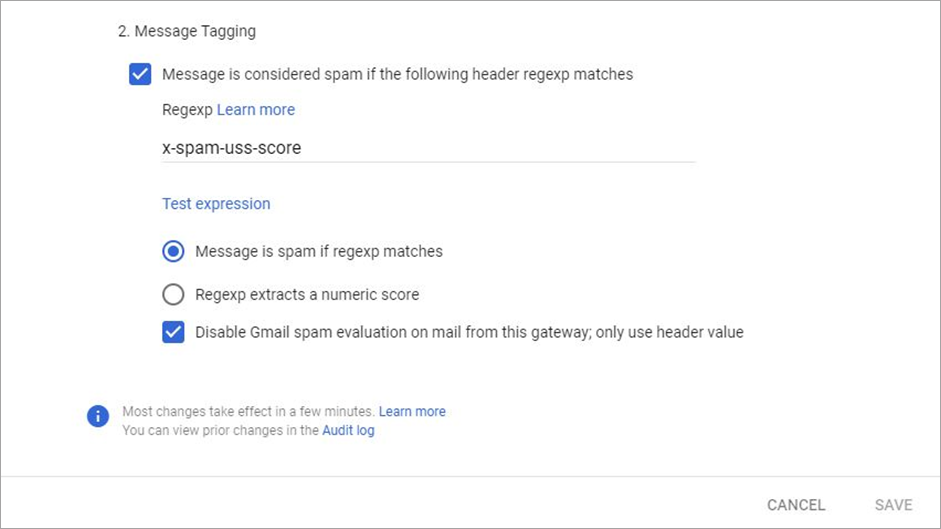The image shows a detailed instruction page set against a white background, centered primarily around the subject of "Message Tagging", denoted as "Number 2". The explanation begins with the text: "Number 2, Message Tagging. Messages are considered spam if the following header, REGEXP, matches." 

Beneath this introductory text, the term "REGEXP" is written out in capital letters twice, followed by a "Learn more" link. 

Following the definition are three distinctive options for handling messages:
1. The first option explains that messages are identified as spam if the REGEXP header matches.
2. The second option suggests that REGEXP can be used to extract a numeric score.
3. The third option offers to disable Gmail's spam evaluation on mail from the specified gateway, using only the header value as a criterion.

At the bottom portion of the page, there is a dedicated interface element combining an icon and supplementary text. The icon is a white circle set within a blue circle. Accompanying this icon is the text: "Most changes take effect in a few minutes." Additionally, there is a "Learn more" link, followed by a sentence indicating that users can review prior changes in the audit log, with "audit log" highlighted in blue, suggesting it is a clickable link.

In the bottom-right corner of the image, there are two final actionable buttons labeled "Cancel" and "Save."